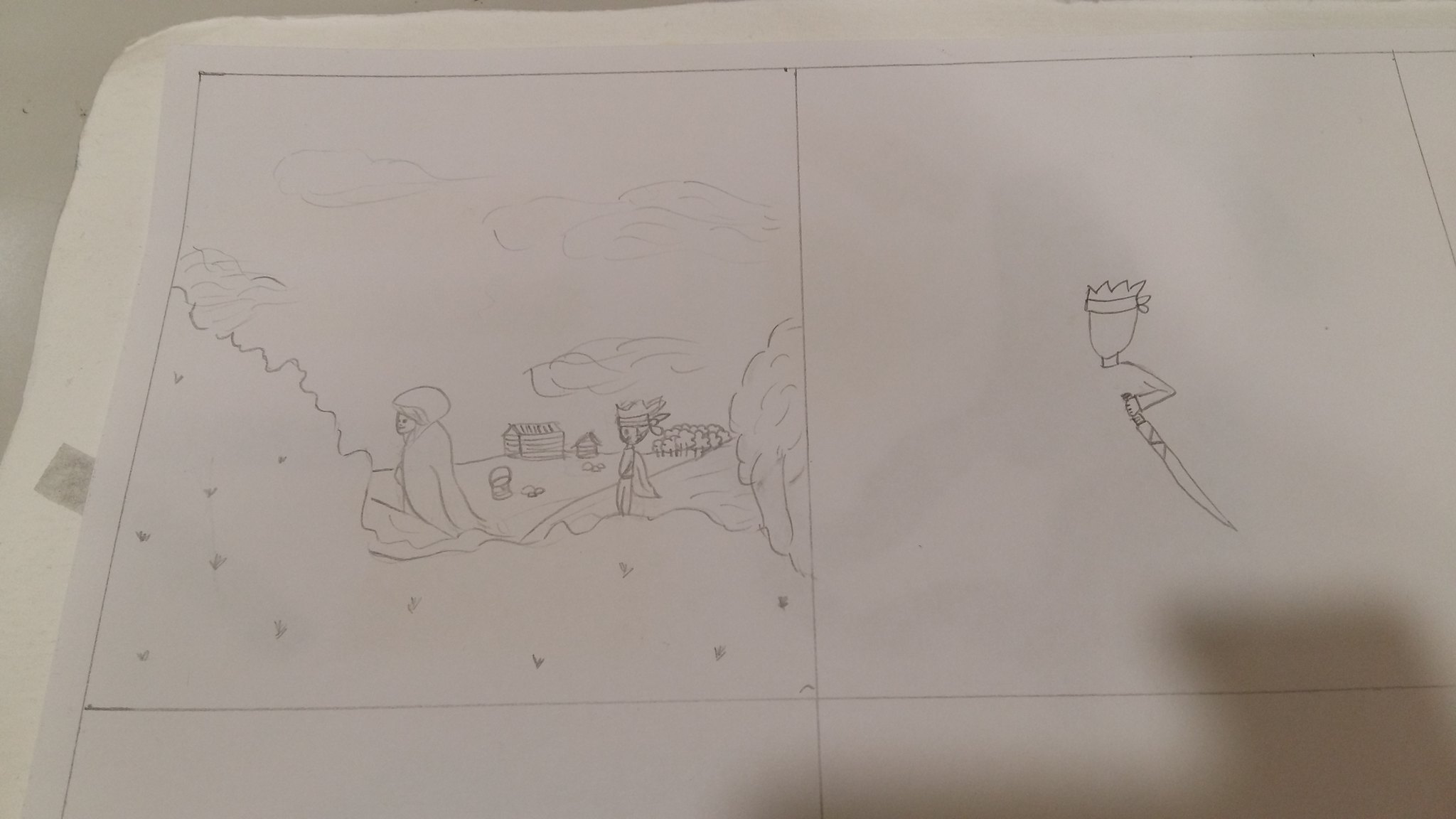This is a detailed penciled art drawing on white paper, meticulously divided into four segments. The upper-left segment features an elaborate scene set outdoors. Here, a woman adorned in robes and a headscarf is depicted sitting on the grass, surrounded by lush greenery and towering trees. The sky above her is dotted with soft, drifting clouds. Approaching from behind her is a man clad in loose clothing and a headscarf tied around his head. His garment flows dramatically behind him as he moves. In the distance, a cluster of trees can be seen, with a rustic log cabin adding to the serene backdrop.

In the upper-right segment, another intricate drawing captures the profile of a man's face. His hair is partially covered by a scarf tied around his head, and although his facial features are absent, a sense of tension is conveyed. His single visible arm is bent at the elbow, gripping a long, narrow sword. The detailed portrayal of his arm and weapon suggests a sense of readiness and anticipation.